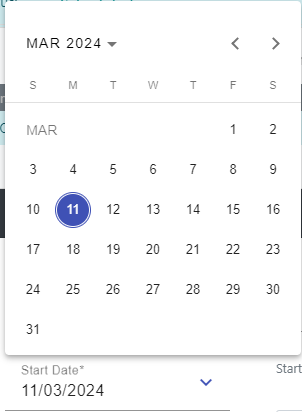This image is a screenshot of a digital calendar page for March 2024. The text "March 2024" is prominently displayed in the upper left-hand corner, alongside a downward-facing arrow that likely indicates a dropdown menu for selecting different months or years. On the far right of this toolbar, there are navigational buttons for moving forward and backward through the calendar.

Beneath the month and year header, the days of the week are listed as "S M T W T F S," representing Sunday through Saturday. A thin gray line separates this header from the calendar grid below. On the left side, the month is abbreviated as "MAR" to align with the grid layout. The calendar spans from the 1st to the 31st, with each day displayed in its corresponding weekday column.

The date "11" is particularly notable, as it is highlighted with a blue circle, making it stand out from the other dates. At the bottom of the page, there is a label that reads "Start Date: 11/03/2024." On the far right side of this bottom section, a button labeled "Start" is visible, suggesting that this is an interactive calendar where users can set or initiate some form of action starting from the selected date.